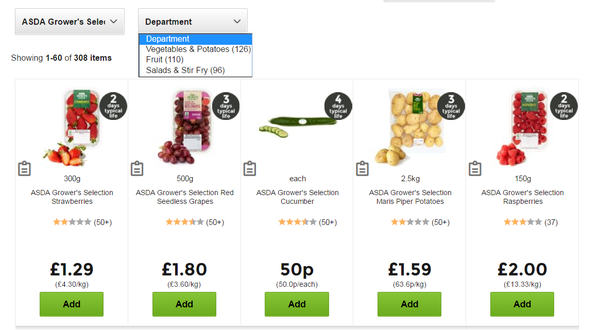This image is a screenshot from an online grocery store, featuring a clean white background. In the upper left-hand corner, a gray rectangle displays the label "ASDA Grower's Selection." To the rectangle's right, the word "Department" appears with a drop-down menu beside it, currently set to display "Vegetables, Potatoes, and Fruit." Just to the left of this dropdown, the text "Showing 1 to 60 of 308 items" is visible.

On this particular page, there are six items shown in a neat, left-to-right arrangement. Each item is presented with a clear and attractive photo, followed by a description, price, and an "Add" button for easy inclusion in the shopping cart.

The first item on the far left is a container of ripe strawberries in an oblong clear plastic package, labeled "ASDA Grower's Selection Strawberries." Below the label, the price is marked at £1.29, and beneath that, a rectangular olive green "Add" button is available.

Next to the strawberries, there is a pack of red seedless grapes, followed by a fresh cucumber. To the right of the cucumber, a bag of potatoes is displayed. Further to the right, a box of vibrant raspberries completes the row. Each item maintains the same format, listed with a clear product image, a descriptive label, and the price along with the "Add" button for simplicity and convenience.